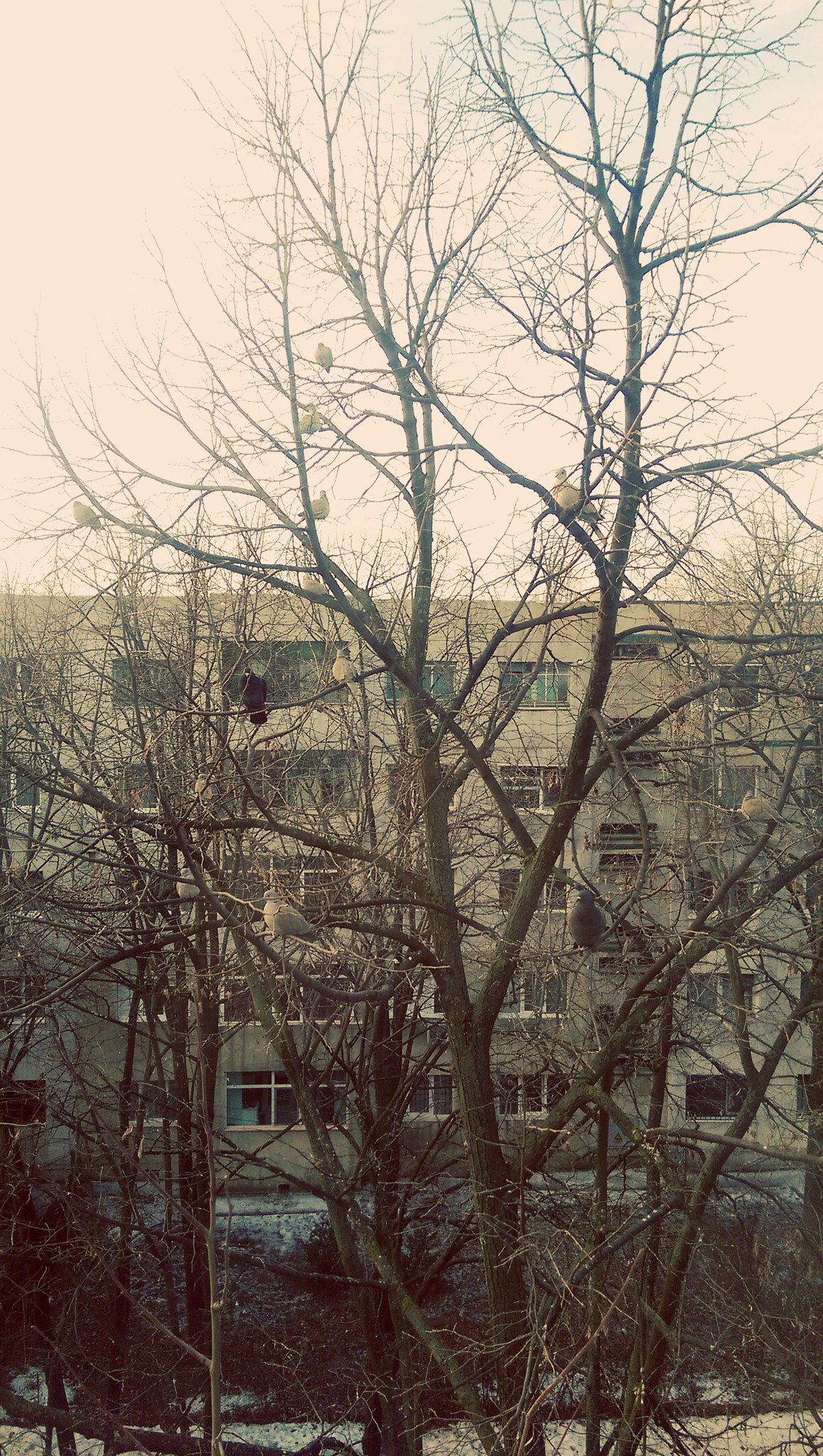This photograph captures a dreary, wintry scene that evokes a melancholic atmosphere. Dominated by a tall, leafless tree with thick brown branches and twigs that appear lifeless, the image's lack of vibrant colors enhances its somber mood. Nestled within the barren tree are about five plump white birds, some appearing to look directly at the camera while others gaze in different directions. The sky in the background is a dull, overcast gray, tinged with a faint pink hue. Beyond the tree stands a beige, Soviet-style apartment building with rectangular windows, its cold, monotonous facade partially obscured by the tree's branches. The snow blanketing the ground confirms the chilly, late-winter setting.